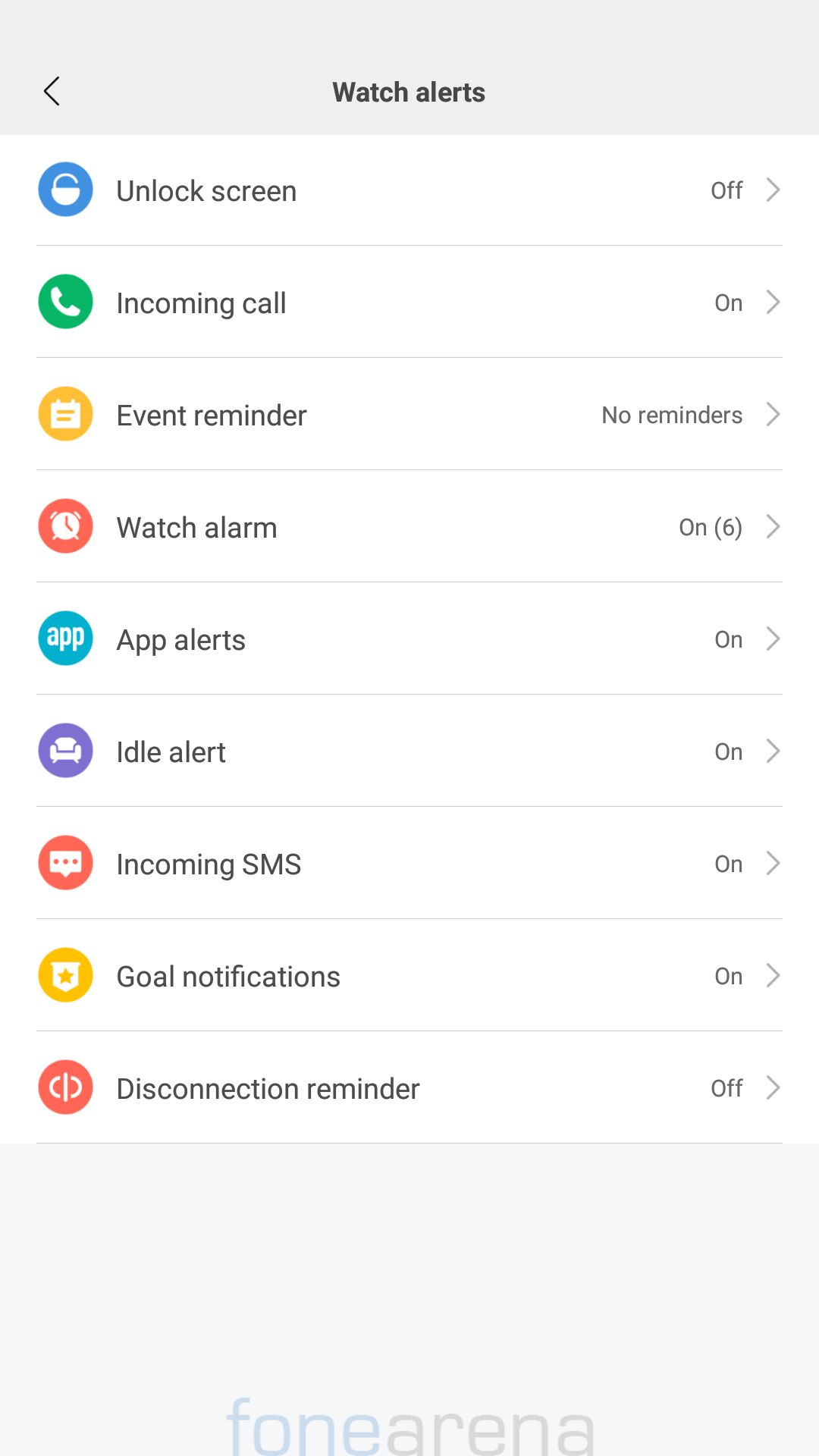The image showcases a user interface screen primarily featuring a white background with a gray header. The header area contains a leftward-pointing arrow and the text "Watch Alerts" in black. Below the header, the layout continues with various settings and their statuses:

1. **Unlock Screen**: Displays "Off" on the right, accompanied by a right arrow.
2. A gray dividing line.
3. **Incoming Calls**: Set to "On" with a right arrow.
4. Another gray dividing line.
5. **Event Reminder**: Displays "No reminders" with a right arrow.
6. A gray dividing line.
7. **Watch Alarm**: Set to "On" with six subsettings indicated within parentheses and a right arrow.
8. A gray dividing line.
9. **App Alert**: Turned "On" with a right arrow.
10. A gray dividing line.
11. **Idle Alert**: Activated "On" with a right arrow.
12. A gray dividing line.
13. **Incoming SMS**: Enabled "On" with a right arrow.
14. A gray dividing line.
15. **Goal Notifications**: Active "On" with a right arrow.
16. A gray dividing line.
17. **Disconnection Reminder**: Set to "Off" with a right arrow.

At the bottom of the layout, there is a gray box, featuring the text "Fone Arena" where "Fone" is highlighted in blue and "Arena" in a darker gray color. On the left side within the interface, multiple colorful icons represent different alert types, including blue, green, yellow, orange, turquoise, purple, and red hues.